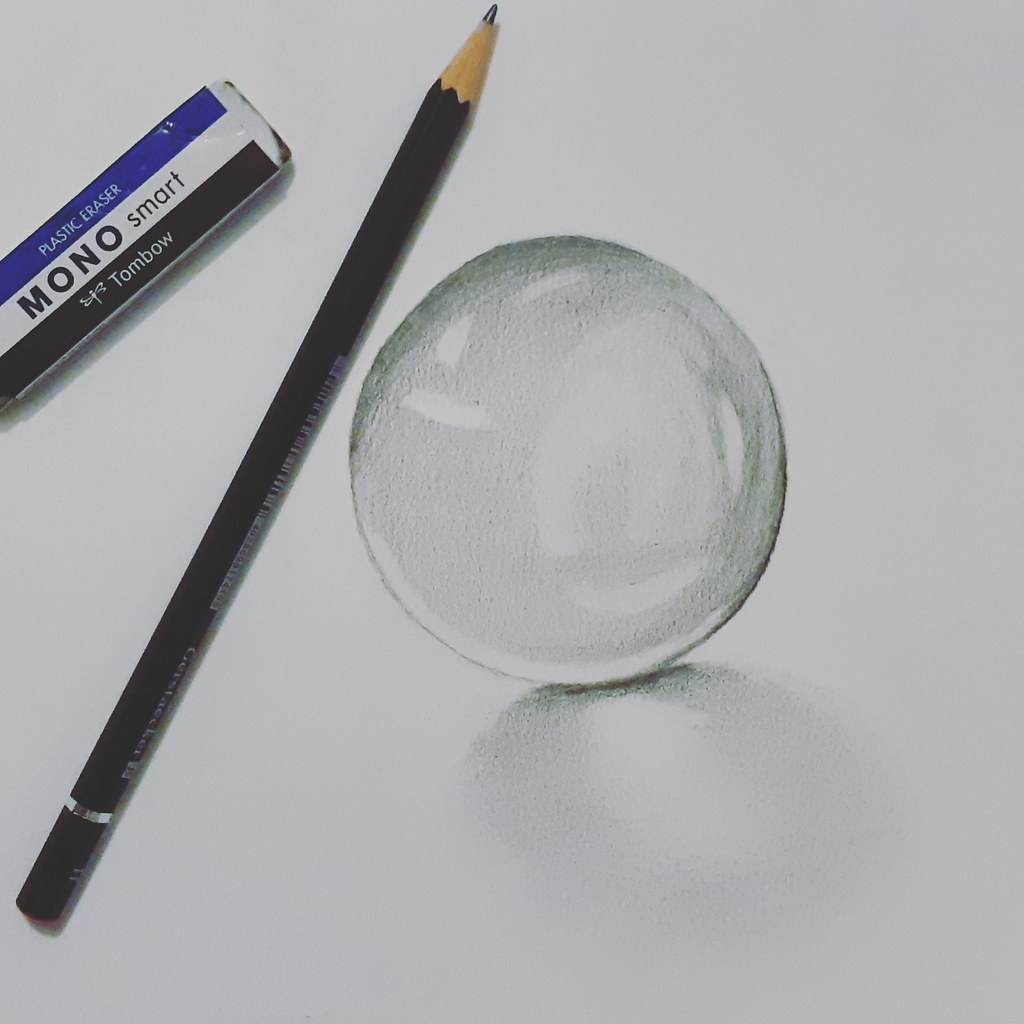The detailed image showcases a carefully drawn pencil sketch of a clear, translucent sphere, possibly representing a glass marble or a piece of ice, positioned at the center of a white piece of paper. The sphere appears to be perfectly smooth, capturing minute details such as having tiny bubbles within it. Diagonally extending from the bottom right to the top middle of the photo, there is a sharpened black pencil with a silver band near the eraser. In the upper left-hand corner of the image, sits a plastic eraser marked "MonoSmart Tombow," identifiable by its packaging with blue, white, and black stripes. The meticulous arrangement and the photorealistic drawing suggest a still-life composition focused on simplicity and elegance.